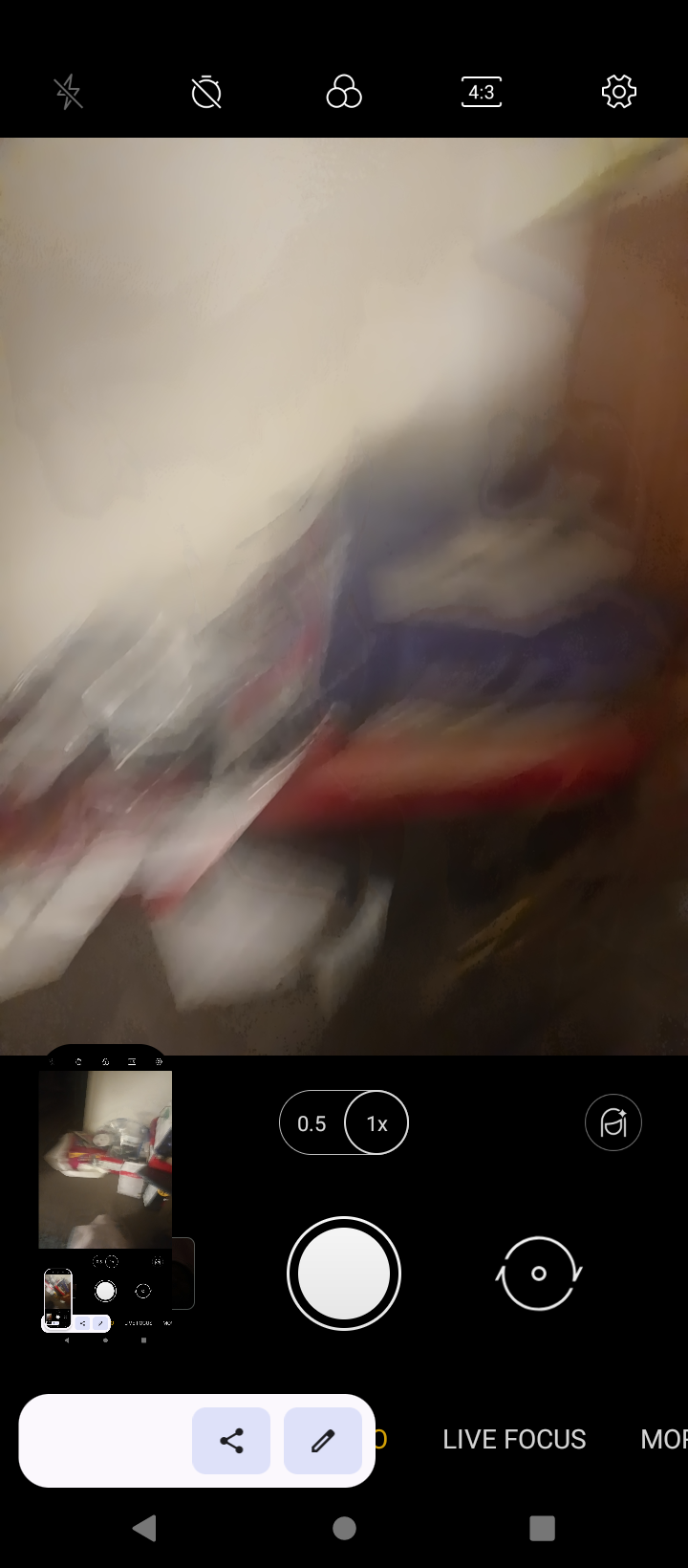A blurry photograph, seemingly taken with a smartphone, is the main subject. The central focus is obscured, making it difficult to interpret, but a white wall and a red table are vaguely discernible, along with some boxes on the table. Notably, the phone appears to have a zoom function set to either 1x or 0.5x. 

In the photo's bottom left corner, there is a smaller, clearer inset image showing the intended subject: a stack of various boxes. This inset image features an array of red boxes, with some having white tops, and others being white with red lids. These boxes are stacked neatly against a white wall on a brown carpet. The orientation and zoom suggest that the phone's camera had trouble focusing, resulting in a poorly zoomed-in screenshot with an aspect ratio of 4:3.